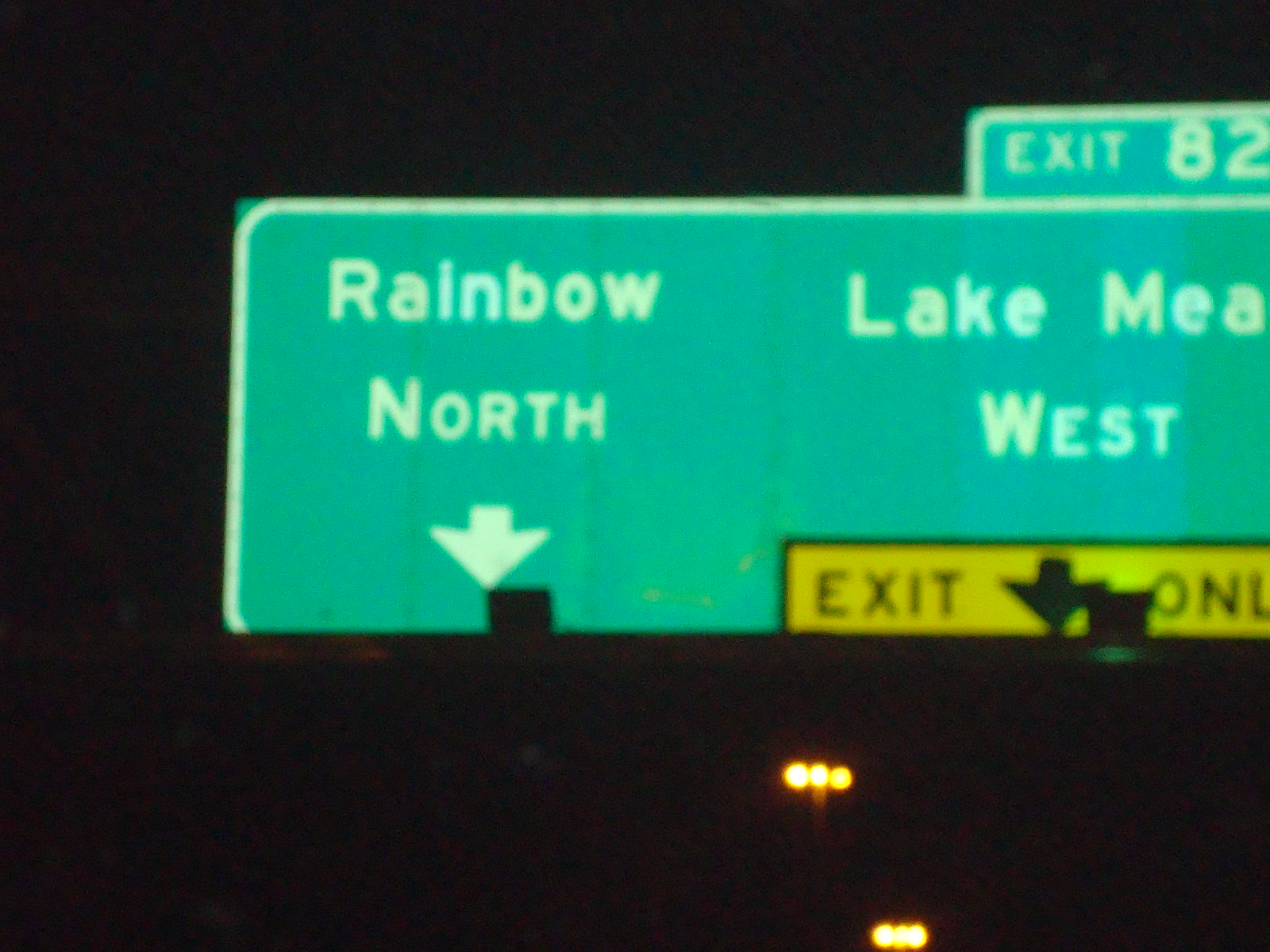This nighttime image depicts a slightly blurry freeway sign illuminated by what appears to be car headlights or streetlights. The large, rectangular sign is bright green with white text and has a white outline. At the top of the sign, "Exit 82" is prominently displayed. Below this, on the left side of the sign, the text reads "Rainbow North" accompanied by a downward-pointing white arrow. To the right, the text "Lake Meadow West" or partially visible "Lake MEA West" is displayed, also accompanied by a downward-pointing arrow. Below these directions, a yellow section is present with the text "Exit Only" in bold black lettering and a black arrow pointing downward, surrounded by a black trim. The sign is mounted on a large pole, and the background is completely black, indicative of nighttime. At the bottom of the image, there are two sets of small, bright yellow lights arranged in three-dot clusters, though they are too blurry to clearly distinguish.